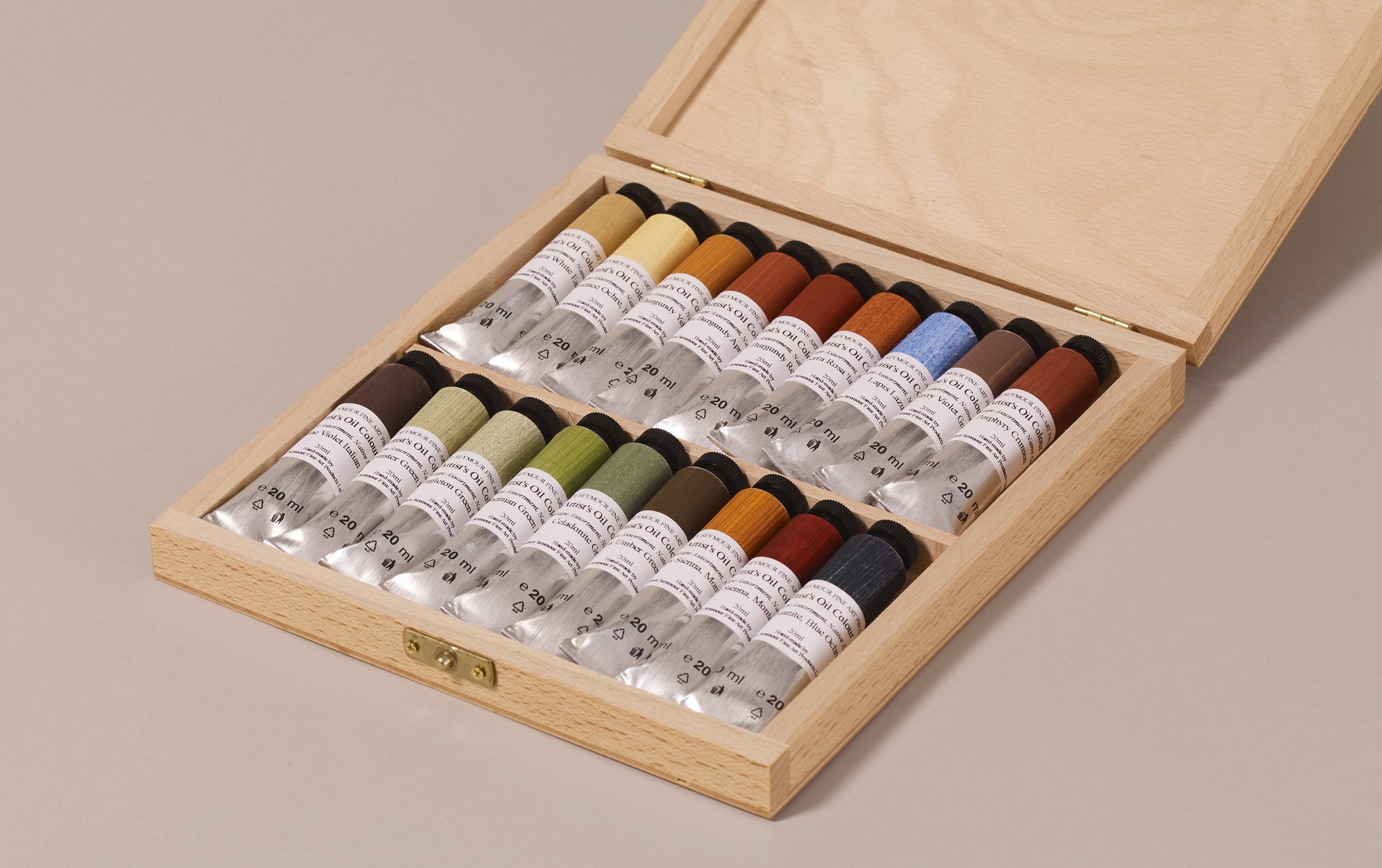The image features a light brown wooden box, open to reveal 18 tubes, likely of acrylic paints, arranged in two rows of nine. The box is shallow with visible hinges, set against a peach-colored background. Each paint tube displays a clear bottom that transitions into a colored top, with hues ranging from gold and mustard yellow to various shades of red, orange, blue, brown, green, and black. The top row consists of colors such as mustard yellow, light yellow, light orange, darker orange, darker red, light blue, brown, and darker reddish brown. The bottom row includes shades of brown, light green, sage green, regular green, darker green, and additional variations of orange, red, and blue. Despite their small print, text labels are visible on each tube.